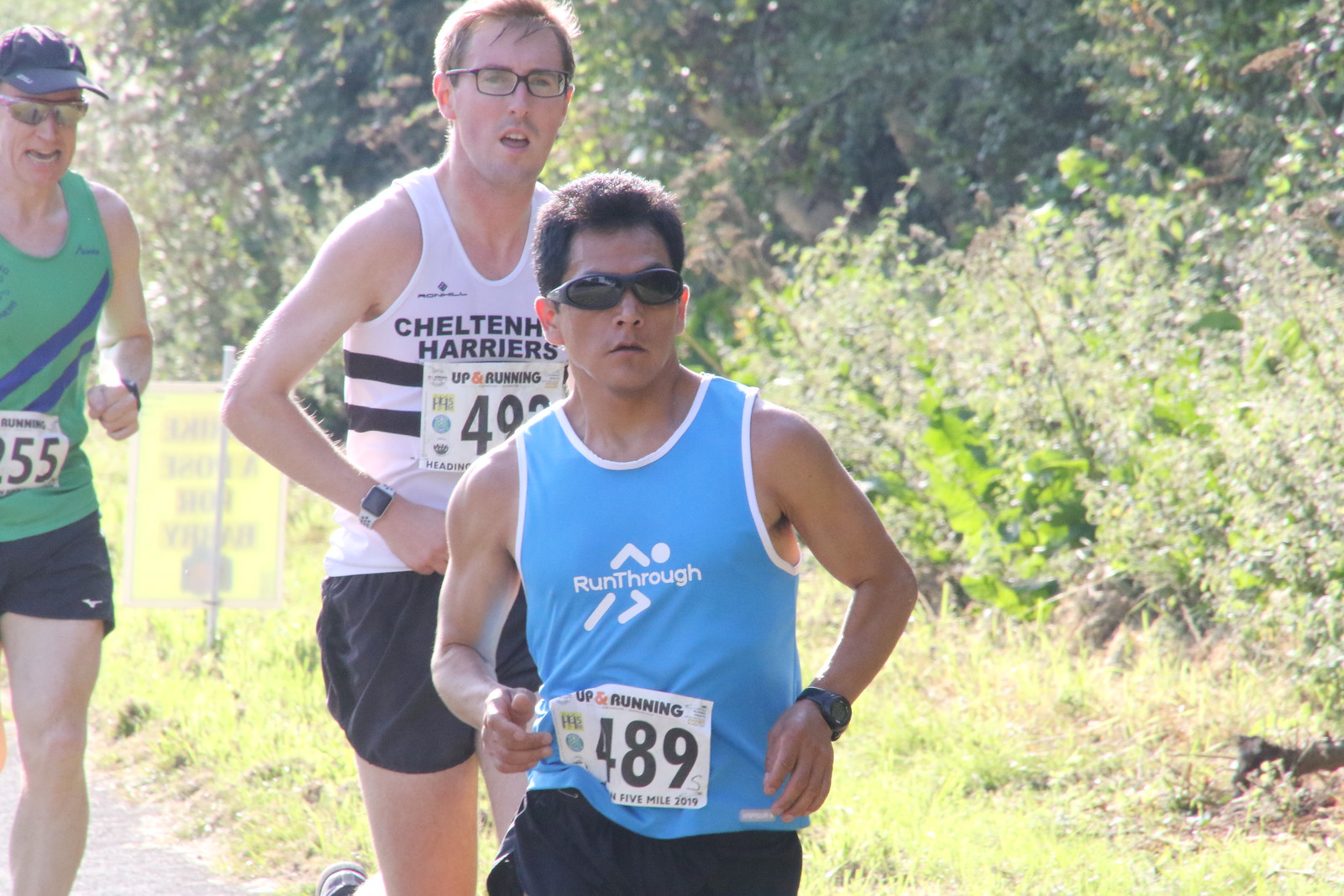Three men are captured mid-stride as they run along a grassy area with trees in the background. The closest runner to the camera is wearing a light blue tank top emblazoned with the words "Run Through" on the front. He accessorizes his athletic outfit with sunglasses, a black sports watch, and black shorts. Close behind him, a taller man is seen sporting a white tank top, black shorts, a watch, and regular glasses. Bringing up the rear, the third runner is dressed in a green tank top and black shorts, complemented by a hat, sunglasses, and a watch. The scene is set against a backdrop of lush green grass and leafy trees, giving it a serene and lively ambiance.